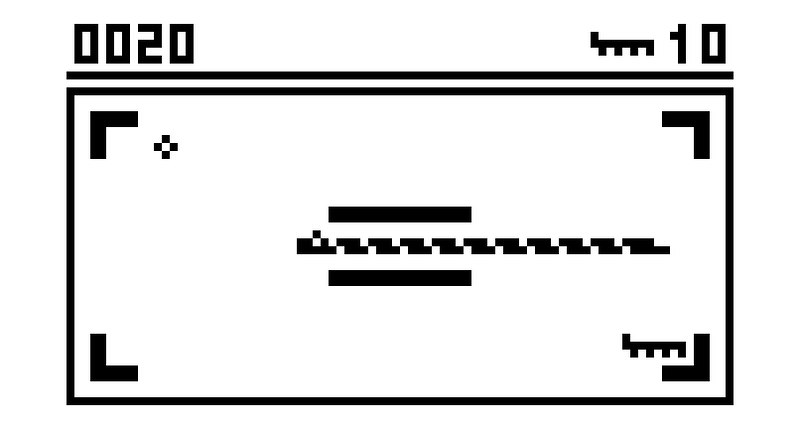This black and white image depicts a screenshot of a very primitive computer game, distinguished by its simple graphical elements and basic score display. The overall format is monochromatic, featuring a stark white background with black lines and shapes defining the layout and game elements. Running along the top edge of the screen are scores displayed in a rudimentary black font, with "0020" on the left side and "10" on the right, hinting at a possible ongoing game or player points.

Beneath the scores, a thick black horizontal line stretches across the screen. Below this line is a large black-outlined rectangle occupying much of the central area, within which the game scene unfolds. Each corner of this rectangle contains an L-shaped black line, oriented with their vertices pointing towards the respective corners, forming a distinctive frame.

In the top left corner of the rectangle, there is a cross-shaped figure composed of four black squares, adding a notable visual element to the game's layout. Centrally positioned within the rectangle are two bold, vertical black lines flanking a pair of longer, serrated black lines, which might represent obstacles or game barriers.

The overall design and graphical simplicity suggest that this image originates from an early era of computer gaming, characterized by its minimalistic and functional aesthetic focused on basic shapes and forms.